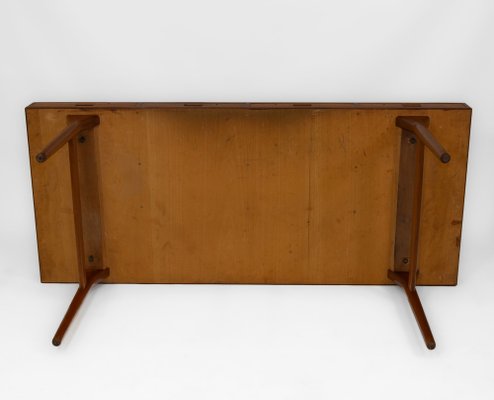The image showcases a wooden table placed centrally on a stark white background. The perspective of the viewer is either from the top looking down or from the side, making it somewhat ambiguous. The table appears to be either on its side or upside down. The table is rectangular in shape and constructed from three joined pieces of brown wood with a distinct grain pattern. Its four legs, slightly darker than the table top, protrude from the edges and have black bolts affixing them to the table. Each set of legs features two bolts, suggesting secure attachment. The table's legs could be made from either wood or metal, although this is unclear due to the image quality. The simplistic white background and lack of any additional elements suggest that this image might be intended for a sales website, emphasizing the detailed structure and form of the table.